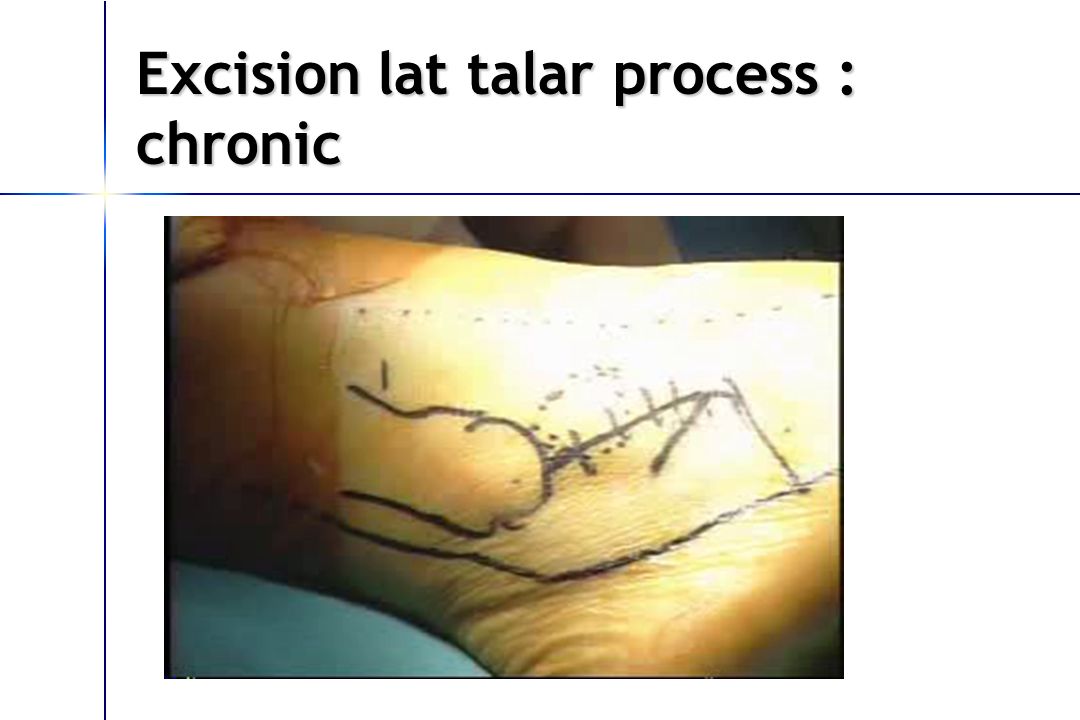The image depicts a detailed surgical diagram centered around a foot, marked with various lines indicating potential incision points. These lines are drawn with precision, suggesting a planned medical procedure, likely in a clinical or hospital setting. The background consists of shades of white and blue, with two blue lines intersecting to form a cross that extends to the edges of the image. In the center of the cross, there's a white glow highlighting the intersection. 

The bottom right quadrant, which takes up a majority of the image, shows the foot section from just above the ankle to a point shortly before the toes. This foot section includes thick black lines on its left and right side and thinner lines on the top and bottom, framing the foot image. The skin is a normal tone, though the ankle area features black markings, some dashed lines and others dotted, indicating where surgical cuts may be made. Additionally, there appears to be a red material, such as a sticker or tape, wrapping around the top part of the foot, likely used to isolate the area for surgery.

Above this image, in the top right quadrant, black text reads "Excision Lat-Talar Process: Chronic," situating the diagram and markings within a specific medical context, likely referring to a chronic condition requiring surgical excision of the lateral talar process. The overall impression is that of an educational medical image designed to guide a specific surgical procedure.